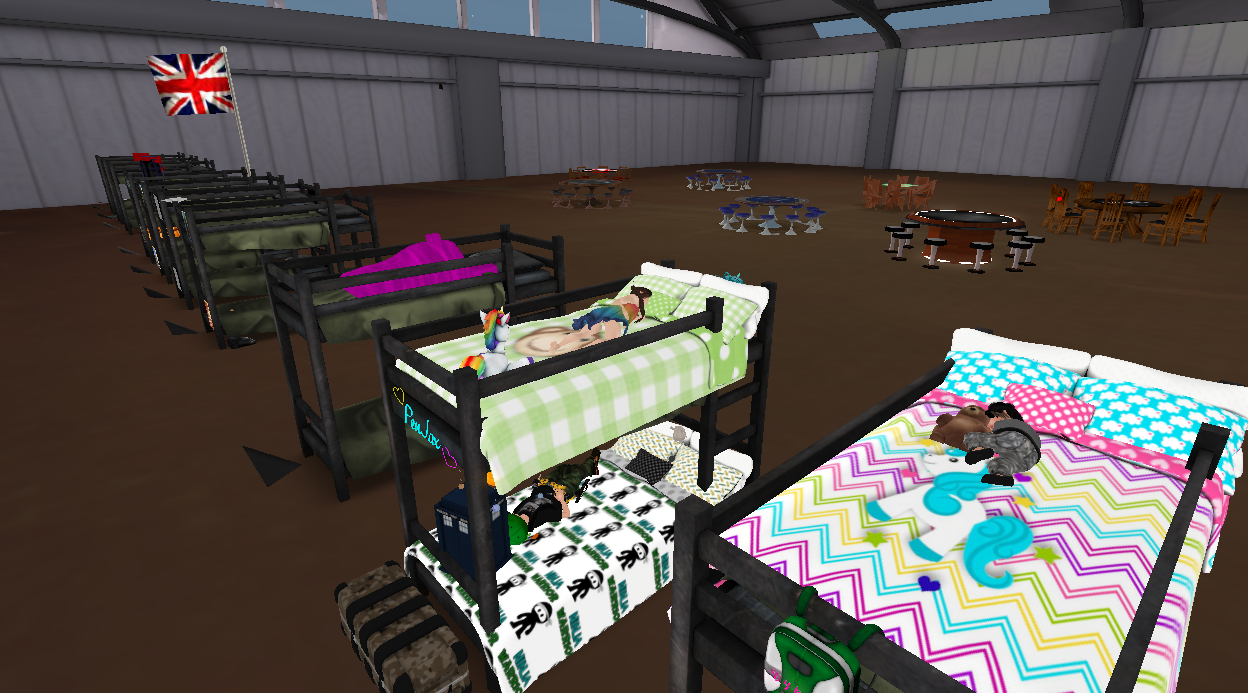The image resembles a scene from a video game, set inside a large, hangar-like structure with greyish walls and large overhead windows revealing a clear, blue sky outside. Prominent in the scene are a series of bunk beds extending from the right side to the left side of the image, each with detailed and colorful bed sheets. One of the noticeable bunk beds features vibrant bedding adorned with a unicorn design, where a child holding a teddy bear is sleeping. Another bed has green and white checkered sheets with a young girl laying on it, next to a stuffed unicorn. There's also a bunk bed with a footlocker displaying white and green lettering and black ninja characters. In the background, a large white flagpole hoists the British flag, identifiable by its red cross and diagonal red stripes. Further into the building, there are circular arrangements of chairs around tables, resembling a cafeteria setting. The atmosphere, while detailed and vibrant, implies a digital world, reinforcing the impression of a scene from a video game.